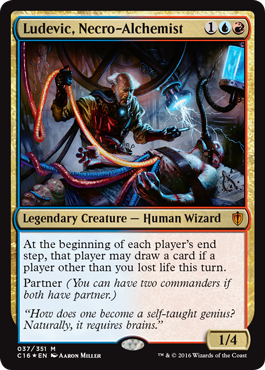The image is a photograph of a Magic: The Gathering card featuring "Ludevic, Necro-Alchemist." The card is encased within an orange and golden border. At the top, the card name, "Ludevic, Necro-Alchemist," is clearly visible. The illustration depicts a bald man with hair on the sides and a beard, who appears to be conducting an experiment on a cadaver lying on a table. Ludevic is holding up a strand of orange cable or entrails, while the pale body on the table has an open torso and is connected to a breathing contraption. Below the illustration, in the card text area, the description reads "Legendary Creature — Human Wizard." The rules text at the bottom of the card states: "At the beginning of each player’s end step, that player may draw a card if a player other than you lost life this turn." Additionally, the card includes the "Partner" ability, allowing the player to have two commanders if both have the partner ability.